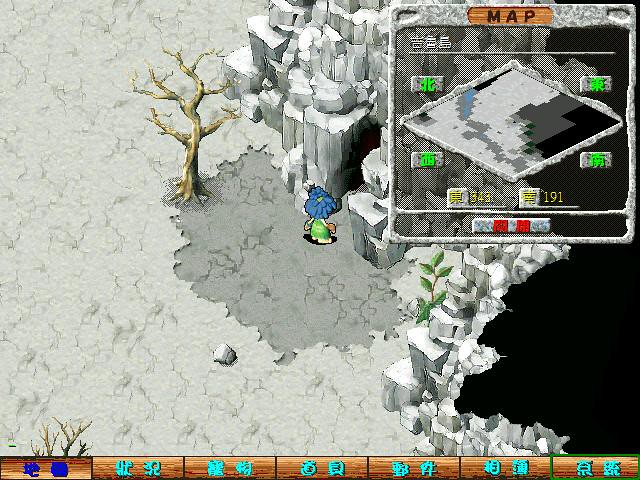In this compelling still image captured from a video game, a character stands poised at the entrance of a foreboding cave. The cave's entrance and the desolate landscape that surrounds it are composed of gray, dry, and crumbly rock, emphasizing a barren and unwelcoming environment. To the right of the cave's entrance, a tree that appears lifeless and devoid of leaves further accentuates the scene’s desolation. In the top right corner of the screen, a map is visible, adorned with various icons that likely indicate points of interest or objectives within the game.

The focal character, noticeably shorter in stature, sports a green shirt and has distinctive blue hair that makes them stand out against the dull backdrop. Along the bottom of the image, a user interface bar displays an array of clickable buttons that resemble wooden planks. Each of these planks is etched with glowing aqua blue characters, suggesting interactive elements that the player can engage with. This detailed setup immerses the viewer in the game's environment, providing a comprehensive overview of both the character and the ominous surroundings they are about to venture into.